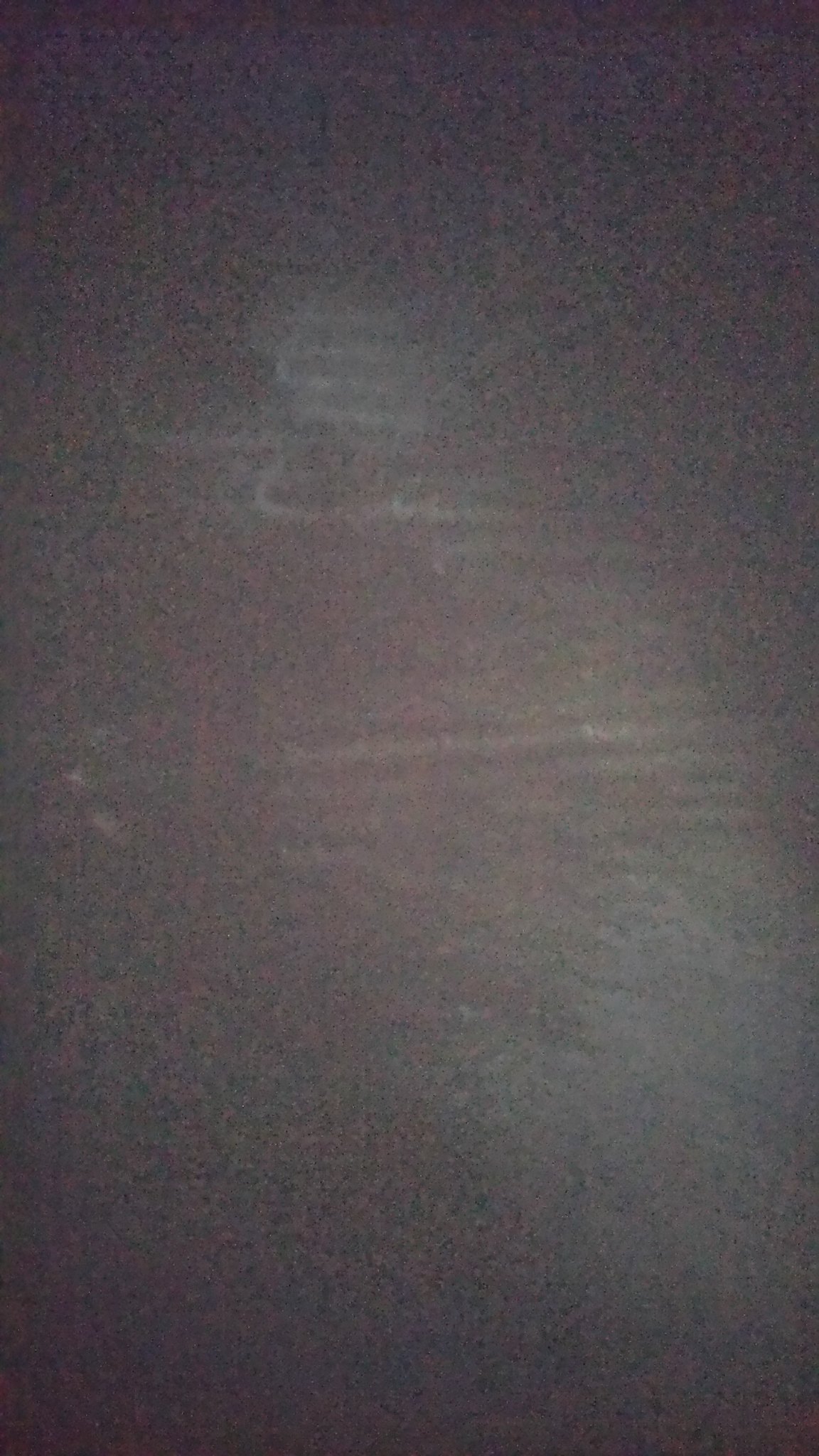This is a tall, rectangular image predominantly featuring a deep black tone. The black backdrop is unbroken without any clear borders, creating an almost solid black canvas. Despite its darkness, the image is marked by a series of blurry, horizontal, and looping lines primarily centered in the midsection. These lines are a mix of white and lighter gray, giving the impression of chalk streaks or smudges. A slight reddish tint appears on the mid-left, subtly coloring the area without fully obscuring the black beneath. The lines weave in and out of the blackness in a staggered pattern, angling and curving from left to right and back again, giving the image a sense of motion and depth despite its graininess. This image has a hauntingly abstract quality, as if captured at night, with indistinct shapes that might evoke something like a shoe print due to the sporadic, blurry streaks throughout.